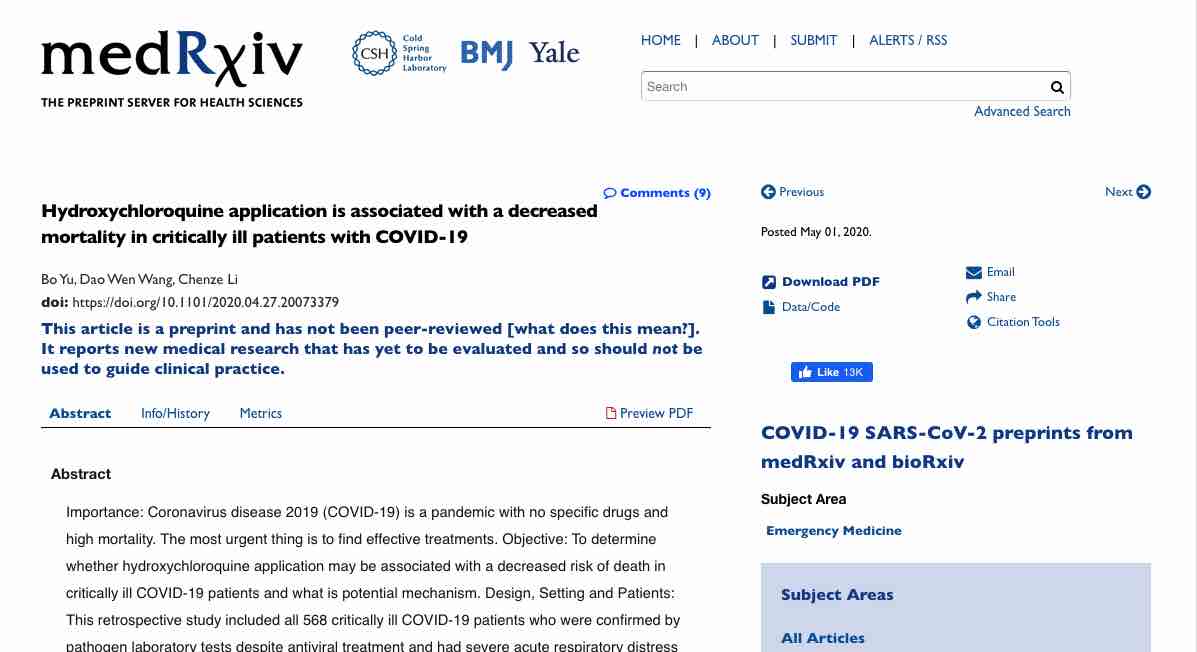A detailed screenshot of a medical website, possibly MyChart or a similar platform, showing a page from MedRxiv. On the top left, the MedRxiv logo is displayed alongside the initials "CSH" encircled. The familiar BMJ blue font and Yale navy blue font can also be seen. The navigation bar contains options such as Home, About, Submit, and Alerts, each separated by vertical dividers. Below, a search bar occupies the space with a black rectangle, and an 'Advanced Search' option is in blue font underneath.

The title of the article, "Hydroxychloroquine Application is Associated with a Degree to More Critically Ill Patients with COVID-19," is prominently featured. A notice clarifies that the article is a preprint and has not undergone peer review; it cautions that the findings are preliminary and should not guide clinical practice. The page offers tabs labeled Abstract, Info/History, and Metrics for further information.

On the right side of the page, details reveal that the article was posted on May 1, 2020. Options to download the PDF, email the article, or share it are conveniently available. The page includes sections dedicated to COVID-19 and SARS-CoV-2 preprints, providing additional information on hydroxychloroquine.